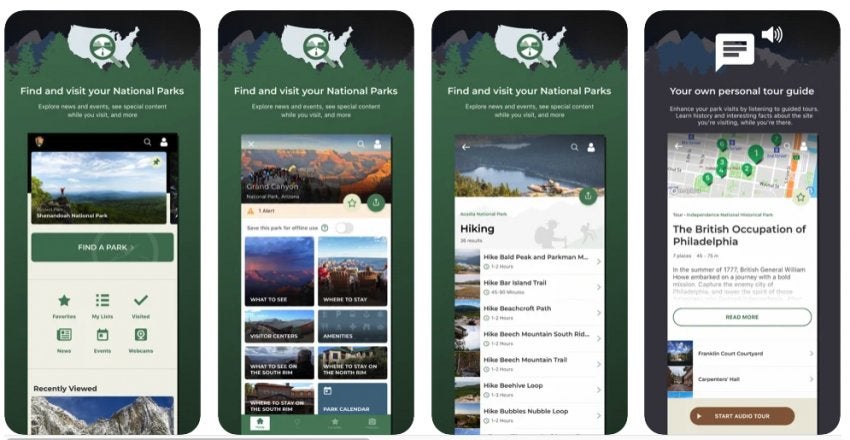The image is a compilation of four different screenshots from an application focused on exploring national parks. Here's a detailed breakdown:

1. The first screenshot features a green background with a black header displaying the text "Find and Visit Your National Parks." It has a search box where users can "Find a Park," along with featured information and a section for "Recently Viewed" parks. Highlighted is a section for the Grand Canyon, presenting options like "What to See," "Where to Stay," and various other visitor resources.

2. The second screenshot shows a similar theme with the "Find and Visit Your National Parks" header. This screen is dedicated to hiking, listing trails such as "Hike Bold Peak," "Pear Mountains," "Hike Trail," "Hiking Path," "Hike Beach Mountain, South Ridge," "Hike Beach Mountain Trail," "Hike Loop," and another loop trail, providing a detailed array of hiking options.

3. The third screenshot continues with the "Find and Visit Your National Parks" theme. This screen specifically highlights "Your Own Personal Tour Guide." The interface features a black background displaying a map annotated with numbers 1 to 4. This section provides information on "The British Occupation of Philadelphia," allowing users to interact by clicking on and highlighting various details to customize their exploration.

Each screenshot offers a focused aspect of the app, either helping users locate parks, find hiking trails, or learn about historical tours, all within a visually consistent interface.